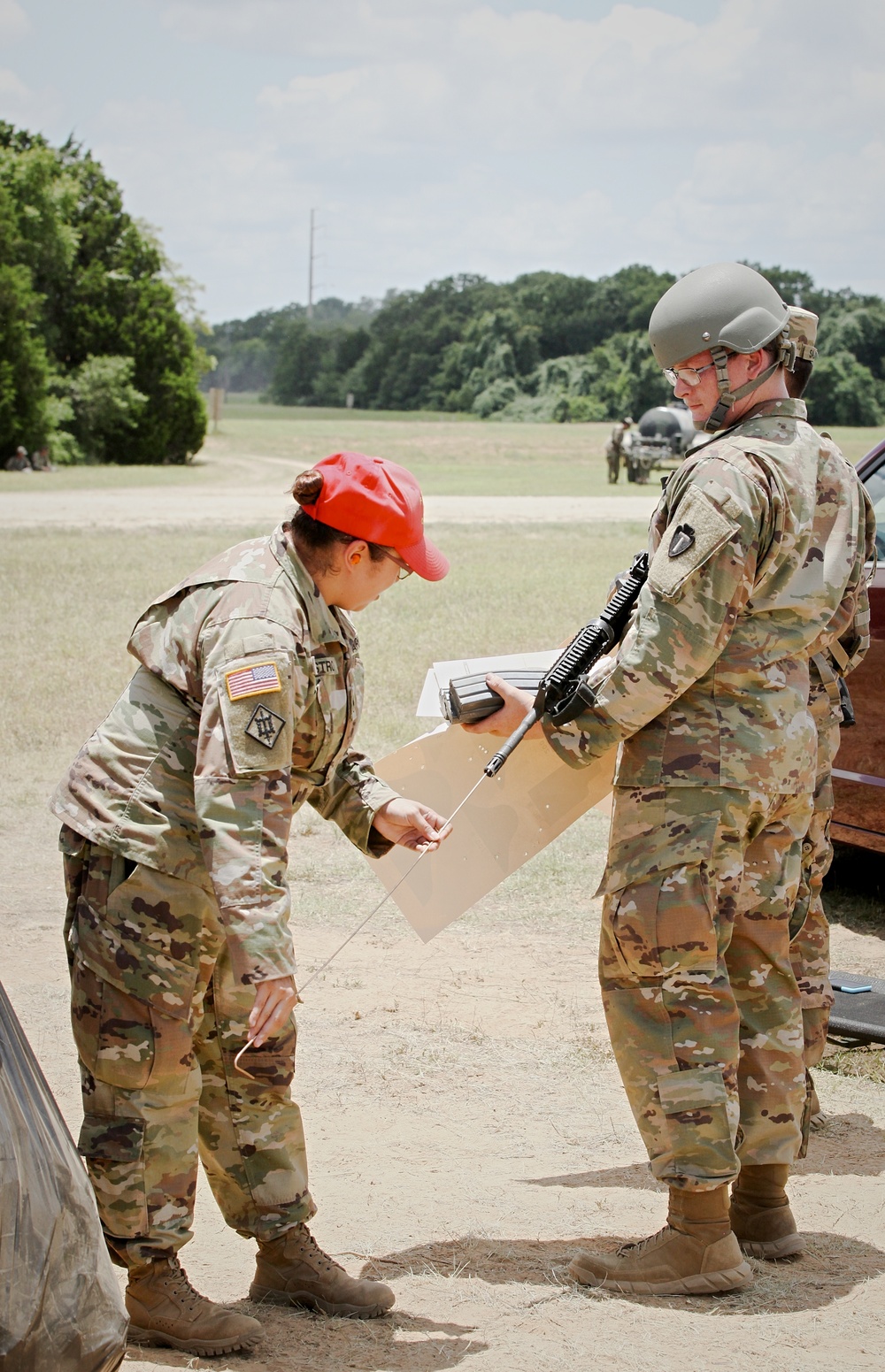The photograph depicts two American military personnel in an open, flat, and somewhat grassy field, with distant trees scattered in the background. Both individuals are clad in official camouflage gear, complete with American flag patches and brown boots, confirming their status as active-duty soldiers. The man, on the right, wears a taupe-colored helmet and glasses and is holding an assault rifle against his right hand and shoulder. The woman, on the left, is identifiable by her red cap and glasses; she appears to be cleaning the barrel of the man's gun using a rod or tube. The man's left hand holds what seem to be schematics and the clips from the gun. In the backdrop, a chopper and another person standing near a black-fronted, white-bodied vehicle add to the authenticity of the setting, suggesting an official military operation. The plain landscape features a road leading towards the vehicle and chopper, underscoring the field training or maintenance task the soldiers are engaged in.